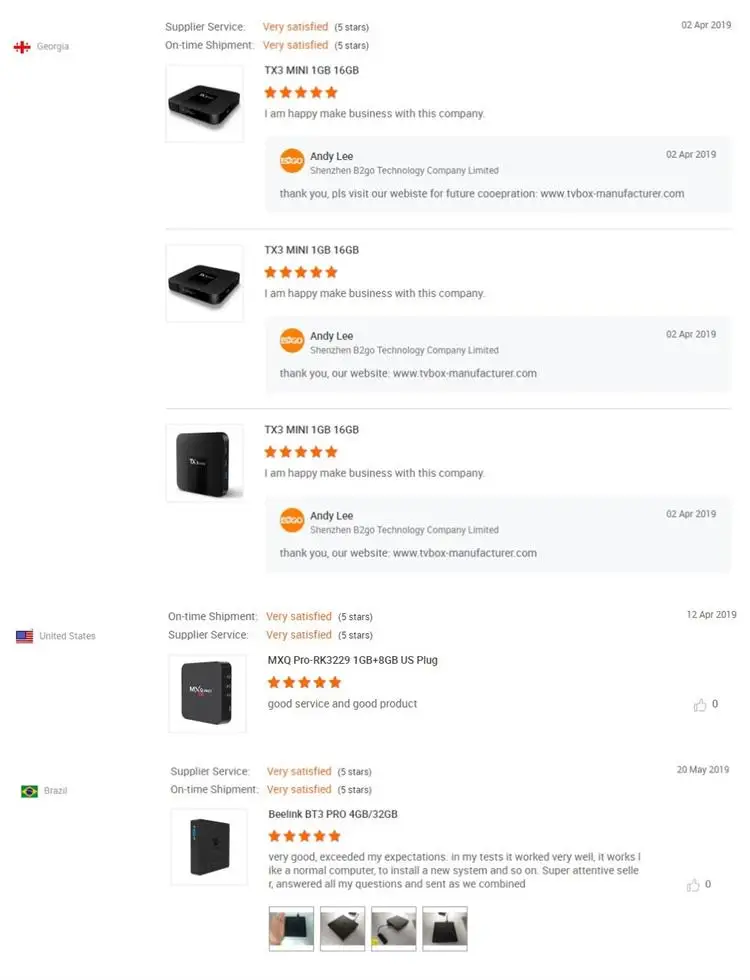**Detailed Description:**

Displayed are various products available for sale, prominently featuring a TX3 Mini Android TV Box. Noteworthy details include a rating system that highlights exceptional service and satisfaction. In the top-left corner, there's an overlay showing a cross symbol with the word "Georgia."

Highlighted customer feedback indicates multiple five-star ratings. Phrases such as "Supplier Service, On-Time Shipment, Very Satisfied," and "Five Stars" emphasize customer satisfaction and timely deliveries. One testimonial reads: "I'm happy you made the business with this company. Andy Lee, Shenzhen B&To-Go Technology Company Limited. Please visit our website for future cooperation: tvbox-manufacturer.com. April 2, 2019."

The testimonials are repeated for different listings of the TX3 Mini, each with specifications of 1GB RAM and 16GB storage, all consistently rated five stars. One entry concludes with: "I'm happy you made business with this company. Andy Lee, thank you. Our website is tvbox-manufacturer.com, dated April 2, 2019."

Overall, the image features five entries of similarly specified TX3 Mini devices, each accentuating high customer satisfaction and endorsements from Andy Lee.